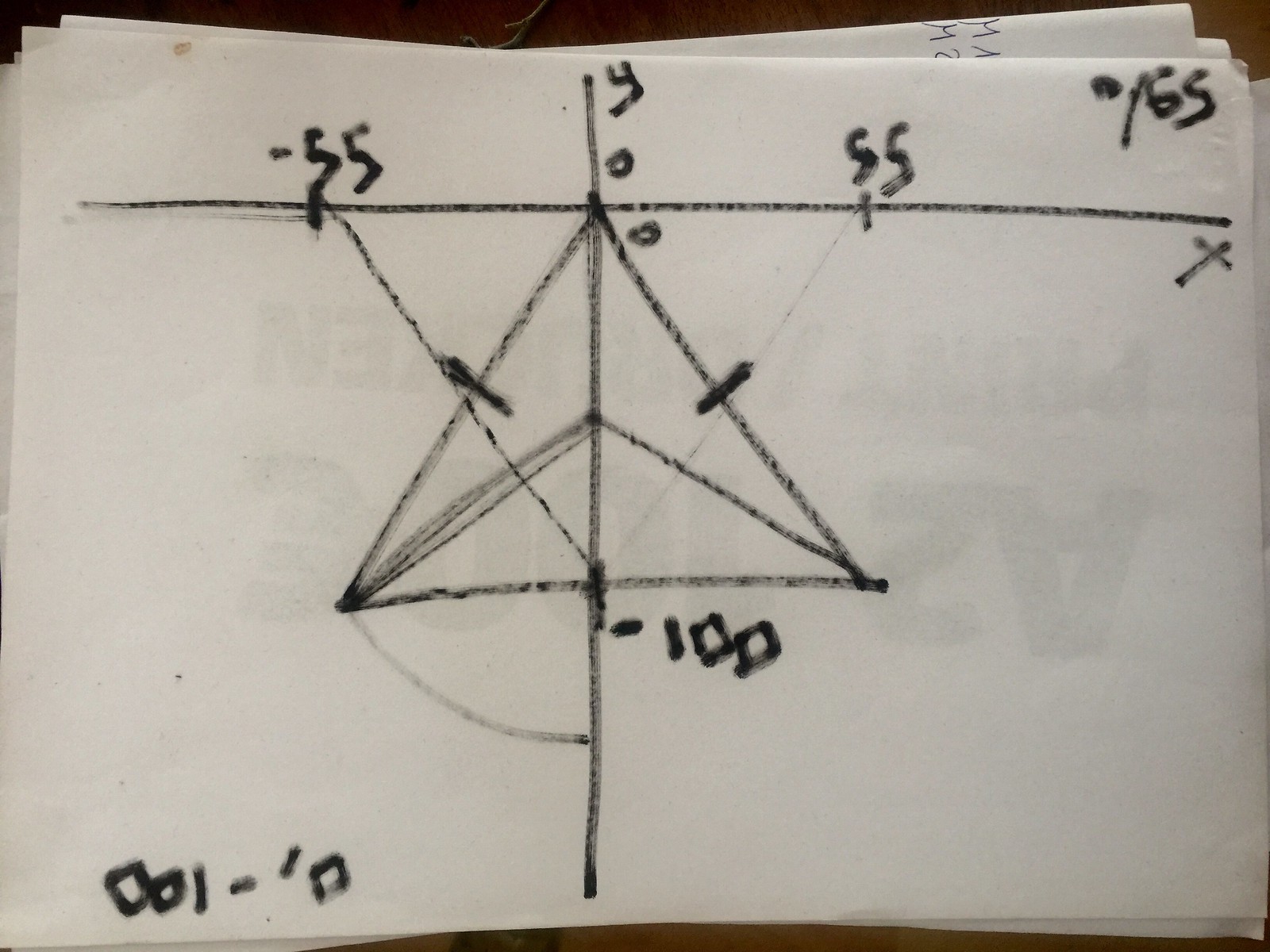This image depicts a rough sketch on what appears to be a napkin or similar piece of paper, part of a stack. Visible through the back of the paper or on the sheet beneath is an upside-down, faded inscription that reads "A to 100 euros print something." 

The main sketch on the forefront illustrates a large lowercase 't', composed of one vertical and one horizontal line intersecting at about 80% of the way up the vertical line. These lines form the axes of a graph, with the vertical line representing the y-axis and the horizontal line, running from -55 to 55, representing the x-axis. 

In the upper right corner, there is a notation stating "0 of 65." The junction of the y-axis and x-axis is marked by a triangle, which contains a smaller triangle within it. At the bottom of the page, an upside-down label indicates "0, -100." 

Overall, this piece of paper features a detailed hand-drawn diagram, suggestive of a conceptual or mathematical representation, overlaid with faded, upside-down text from another source.